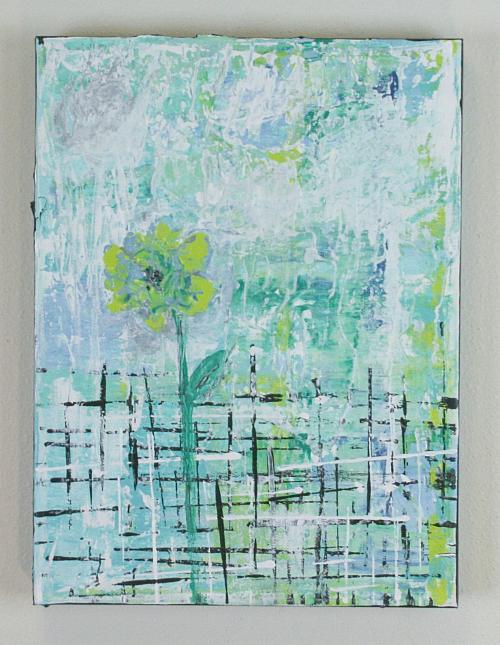This expressive painting, reminiscent of watercolors, is mounted unframed on a white wall, casting a pronounced shadow behind it. The artwork features a single prominent yellow daffodil with a green stem and one leaf, set against a dynamic, abstract background. The daffodil is depicted behind a hatch-mark fence, with vertical and horizontal black lines that suggest garden imagery. The background blends shades of teal, green, blue, and white, resembling a watery sky. The painting extends edge-to-edge, adding to its immersive quality, and a light white wash subtly overlays the vibrant colors. The daffodil serves as the focal point, drawing attention with its bright hue and bold presence amidst the abstract surroundings.